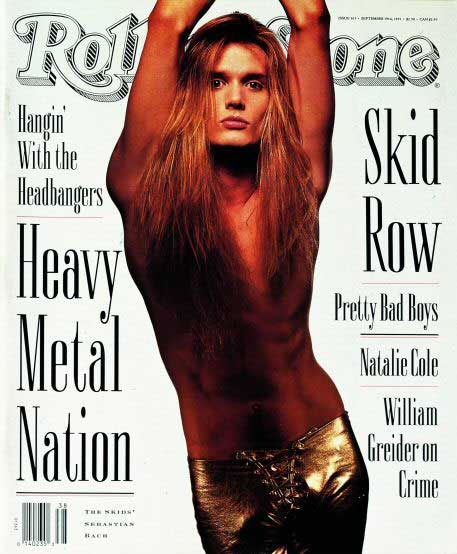This black-and-white Rolling Stone magazine cover features a shirtless white male rock star with long brown hair standing at the center, arms raised above his head. He is wearing gold pants that appear to lace up in the front. The magazine text includes "Rolling Stone" across the top, "Hanging with the Headbangers, Heavy Metal Nation" on the left side, and "Skid Row, Pretty Bad Boys, Natalie Cole, William Greider on crime" on the right side. The cover's primary colors are black, white, gray, tan, and gold, with the man prominently positioned against the backdrop of the magazine's bold text and imagery.